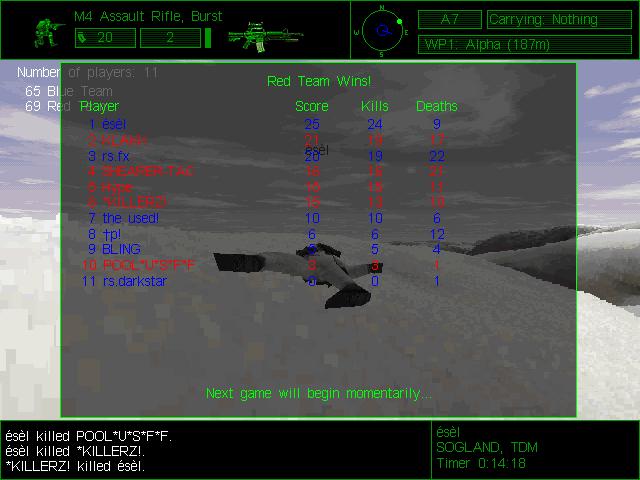A grayscale screenshot from a video game, where the player's character is deceased, is overlaid with various interface elements. Dominated by a monochrome backdrop, the screen features a prominent in-game menu. The top of the menu proclaims the victory of the "Red Team," accompanied by an announcement in green text: "The next game will begin momentarily." Detailed statistics populate the ensuing segments, listing player names, their respective scores, kills, and deaths. Along the bottom and top edges, black borders frame the image, enclosing additional gameplay information.

To the right, the interface displays the player's arsenal, highlighting the equipped weapon: an M4 assault rifle configured for burst fire, along with a directional compass. The bottom-right corner showcases the player's username, "Isil." On the left side, the game logs recount recent events: "Isil killed Poole," "Yusif," and "Isil killed Killers," followed by, "Killers killed Isil." This richly detailed caption encapsulates the intensity and statistical depth of the post-match summary screen.